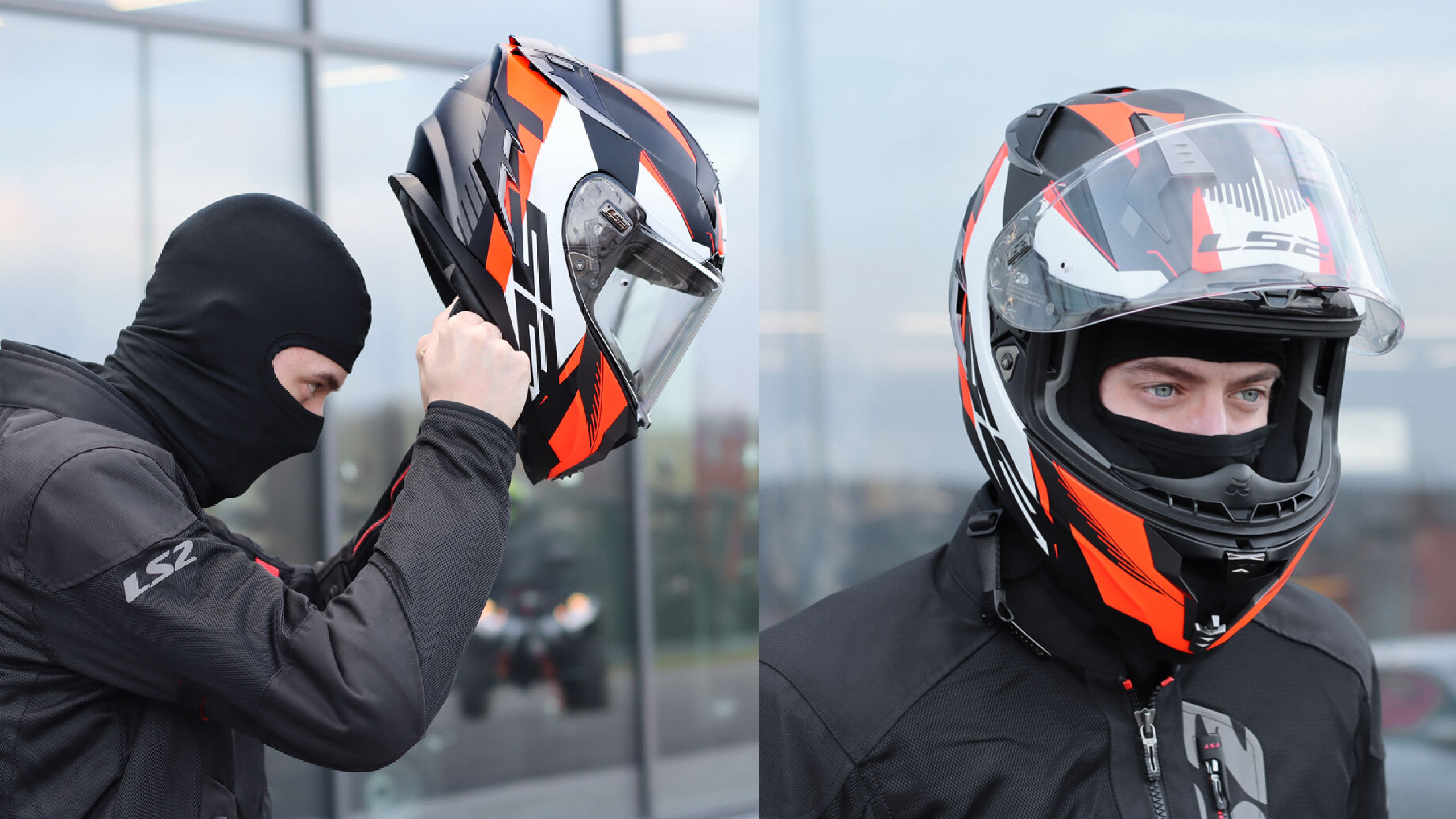In this landscape-oriented photograph, which is divided into two adjacent images, we see the same Caucasian man in both frames, seemingly preparing for a ride. In the left image, the man is shown in profile, his right side visible as he holds a black helmet with orange, white, and black accents, about to put it on. He wears a black ski mask, revealing only his eyes, a black jacket with a silver "LS2" label on the right armband, and stands against the blurred backdrop of a glass building. In the right image, the man, now wearing the helmet, looks slightly to the right, showcasing his piercing blue eyes through the visor. The helmet, same in design as in the left image, complements his black jacket which is zipped up to his neck. The overall setting appears to be daytime, and both images combine to portray the meticulous process of gearing up for a ride, whether it be on a motorcycle or an ATV.